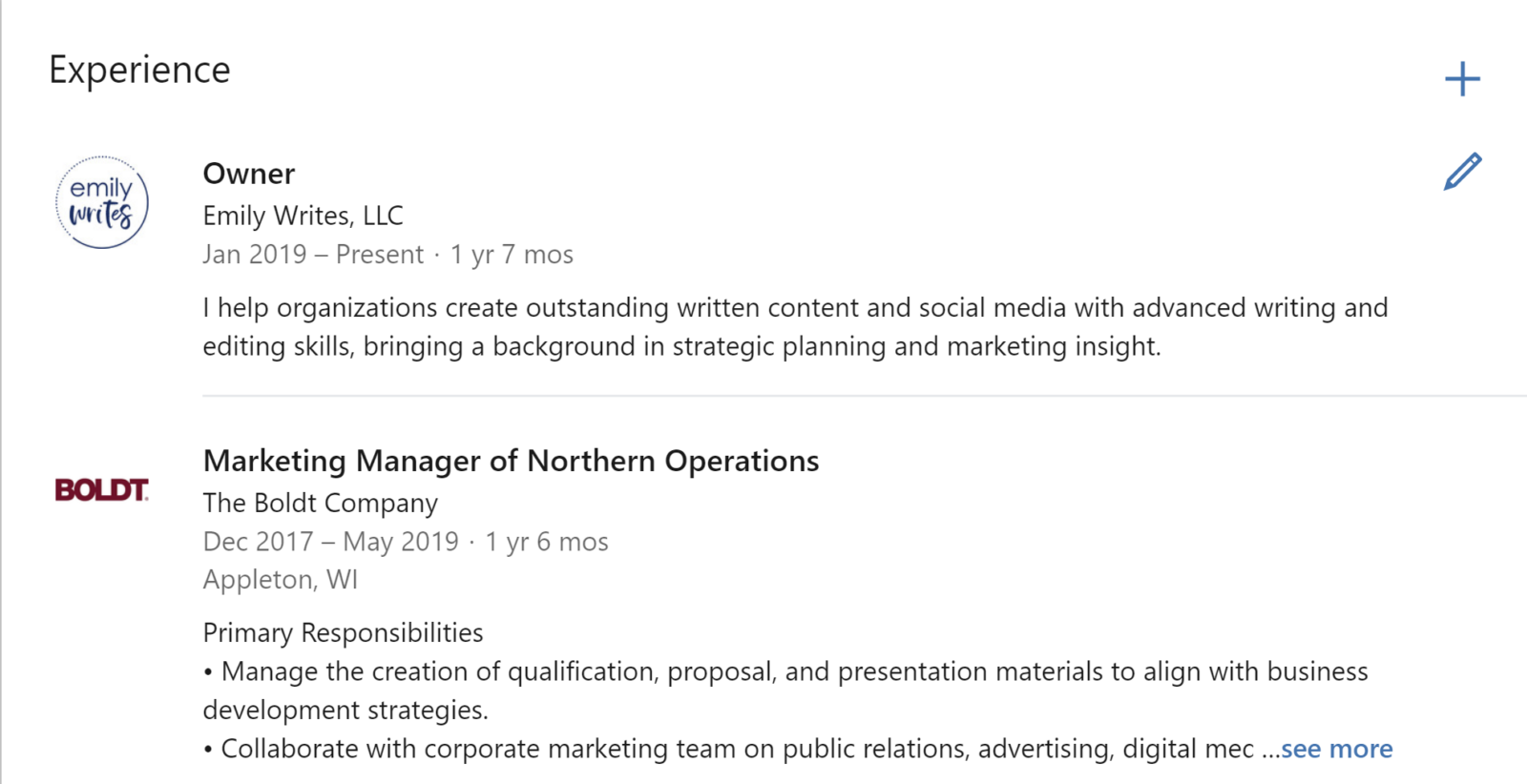This screenshot showcases a section of a professional resume against a clean, white background with black text. Titled "Experience" at the top, the section begins with the logo and position for Emily Wrights, LLC. Emily Wright is noted as the Owner of Emily Wrights, LLC, from January 2019 to the present, spanning one year and seven months. The description highlights her role in helping organizations craft exceptional written content and social media, leveraging her advanced writing and editing skills alongside strategic planning and marketing insights.

Following that, the resume features an icon representing BOLDT and details her position as Marketing Manager of Northern Operations for The Bolt Company from December 2017 to May 2019, a total of one year and six months. Located in Appleton, Wisconsin, her primary responsibilities included managing the creation of qualification, proposal, and presentation materials to support business development strategies. She also collaborated with the corporate marketing team on public relations, advertising, and digital messaging, although the text trails off with “see more” indicating further details available.